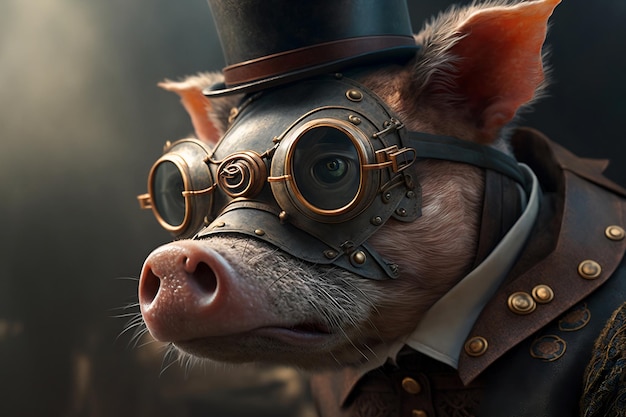The image features a meticulously detailed, steampunk-inspired, computer-animated or CGI pig. This pig, with a pinkish hue and white accents around its snout, sports a pair of distinct black goggles with brass or gold rims around the eyes. He wears a black top hat, the upper part of which is not visible. The pig is dressed in a well-tailored black jacket accented with gold buttons, and it appears to have leather trim around the top edges. Beneath the jacket, a hint of a white shirt with a collar is visible. The attire gives off a vintage, military vibe. The background is blurry, with varying shades transitioning from dark brownish-gray to tan, making the pig the clear focal point.